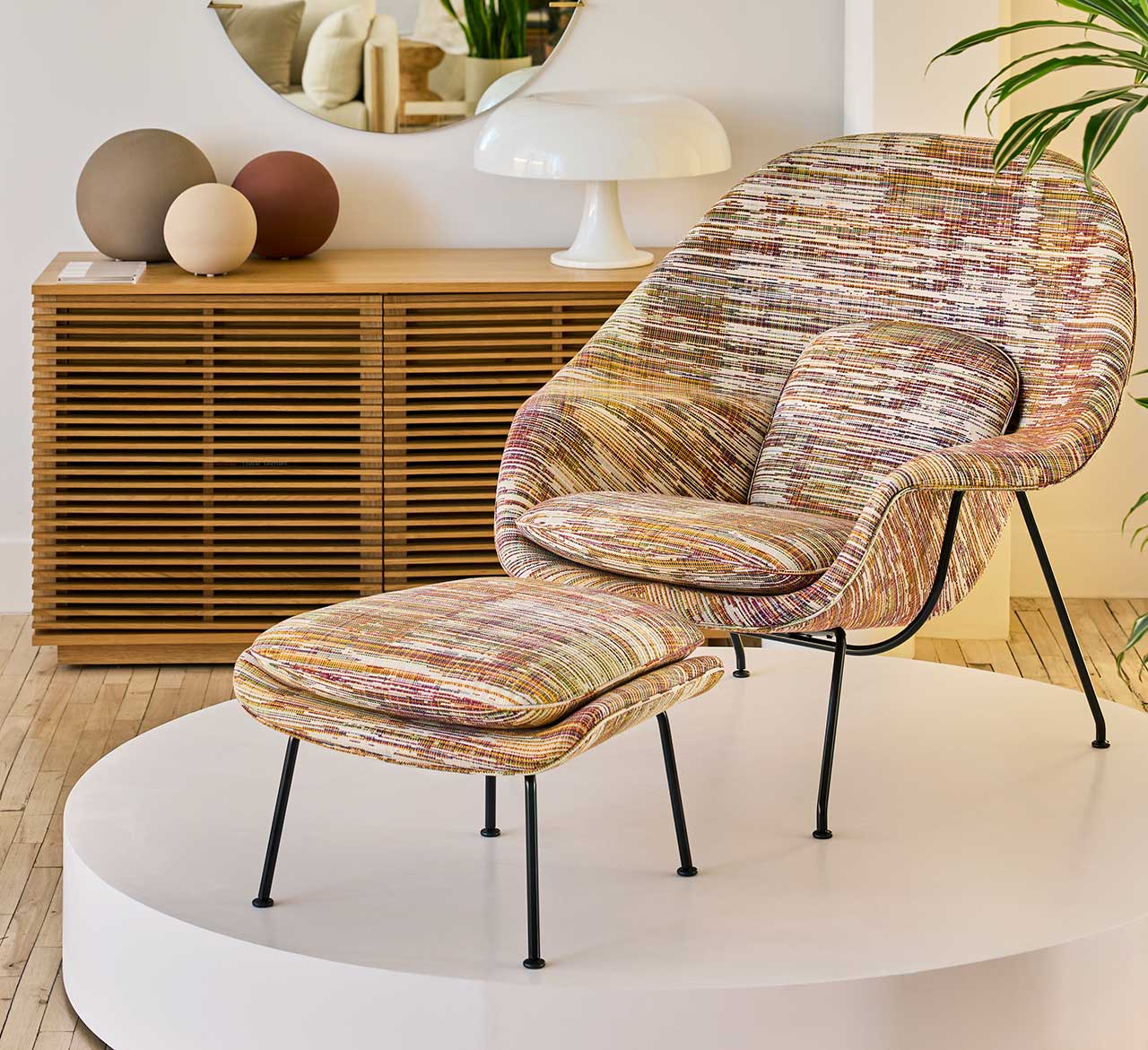The image depicts a cozy living room featuring a uniquely colorful chair and matching ottoman, both positioned on a small, white circular platform that rests on a light brown wood plank floor. The chair has a low, laid-back design, perfect for leisurely activities like reading. It features a metal frame with black legs, and its cushions are adorned with thin vertical stripes in a vibrant mix of pastel colors: white, light brown, dark brown, dark red, and even hints of dark yellow. The cushions are built in and include a square backrest with an oval-shaped back support. Directly in front of the chair is a matching footstool.

In the background, there is a white wall with a wooden cabinet that has a decorative grill front and supports a wide white lamp with a lampshade resembling a mushroom. Additionally, the cabinet showcases a decorative arrangement: a cake plate and three differently colored balls—brown, light brown, and dark red. Above the cabinet hangs an oval-shaped mirror, adding a touch of elegance to the space. The detailed elements and cohesive color palette create a warm and inviting atmosphere in this living room.